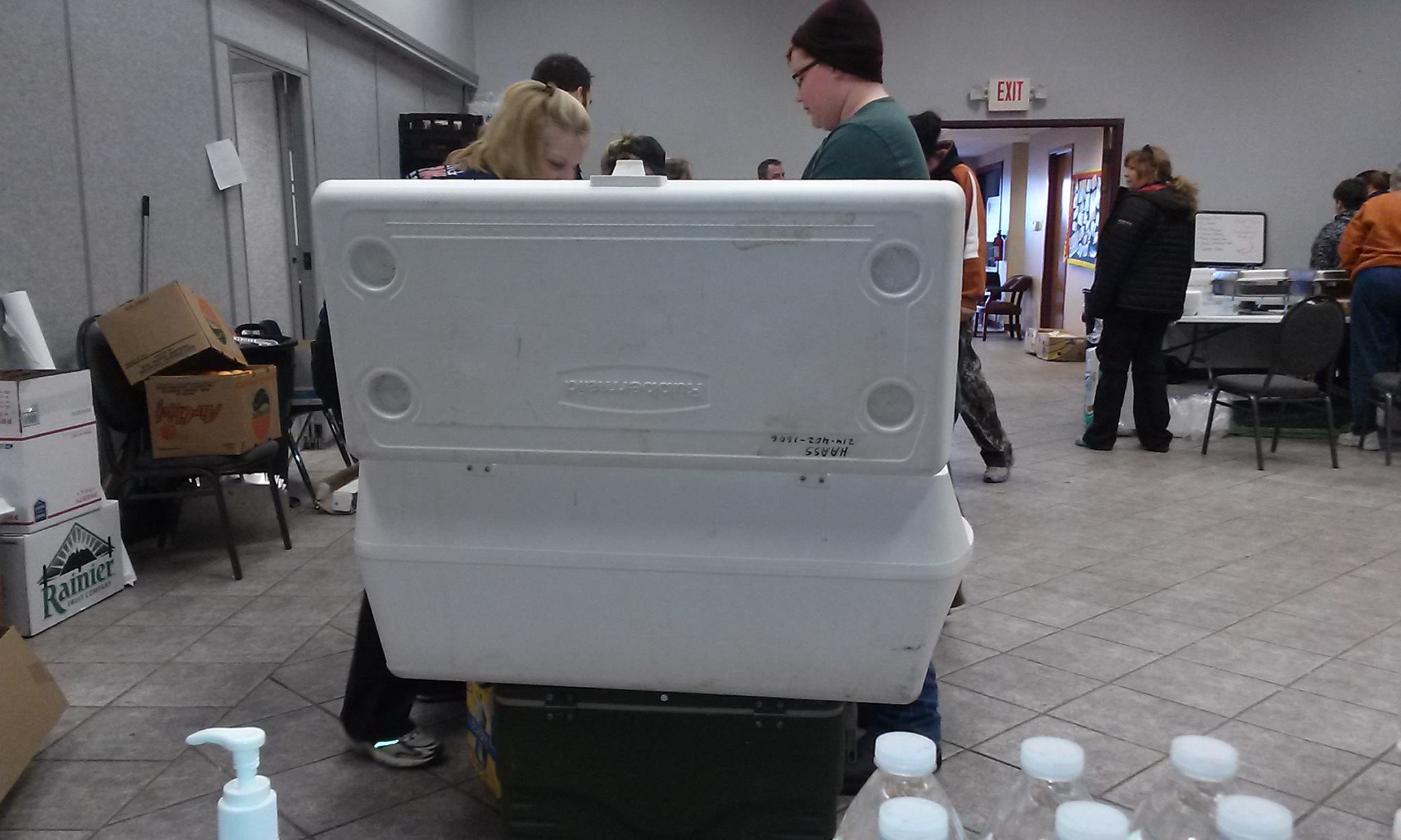The image captures a bustling gathering inside a large room, possibly a conference room or school auditorium. The floor features diagonally laid grayish-brown tiles, except for the outer three to four rows near the dark gray bottom walls, which are parallel to the walls; the upper portions of the walls are a lighter gray. In the distance, a wide door is topped by an unlit exit sign with red letters. Central to the photograph is a white rectangular Rubbermaid cooler with an open lid that has four cup holders integrated into its corners. Beneath it is a smaller black cooler. People are milling about, seemingly setting up for an event. 

In the upper left of the cooler, a blonde woman with shoulder-length hair wearing long black pants is bent over the table, while a man in a green shirt and black skully cap appears on the right edge of the cooler. Scattered throughout the room are people dressed in casual clothing, including black jackets and orange shirts. The foreground shows six clear plastic bottles with white caps arranged near a white hand pump, likely a sanitizer dispenser. On the left side against the wall are brown boxes and chairs, with a box labeled "Rainier" at the bottom of a stack of white boxes.